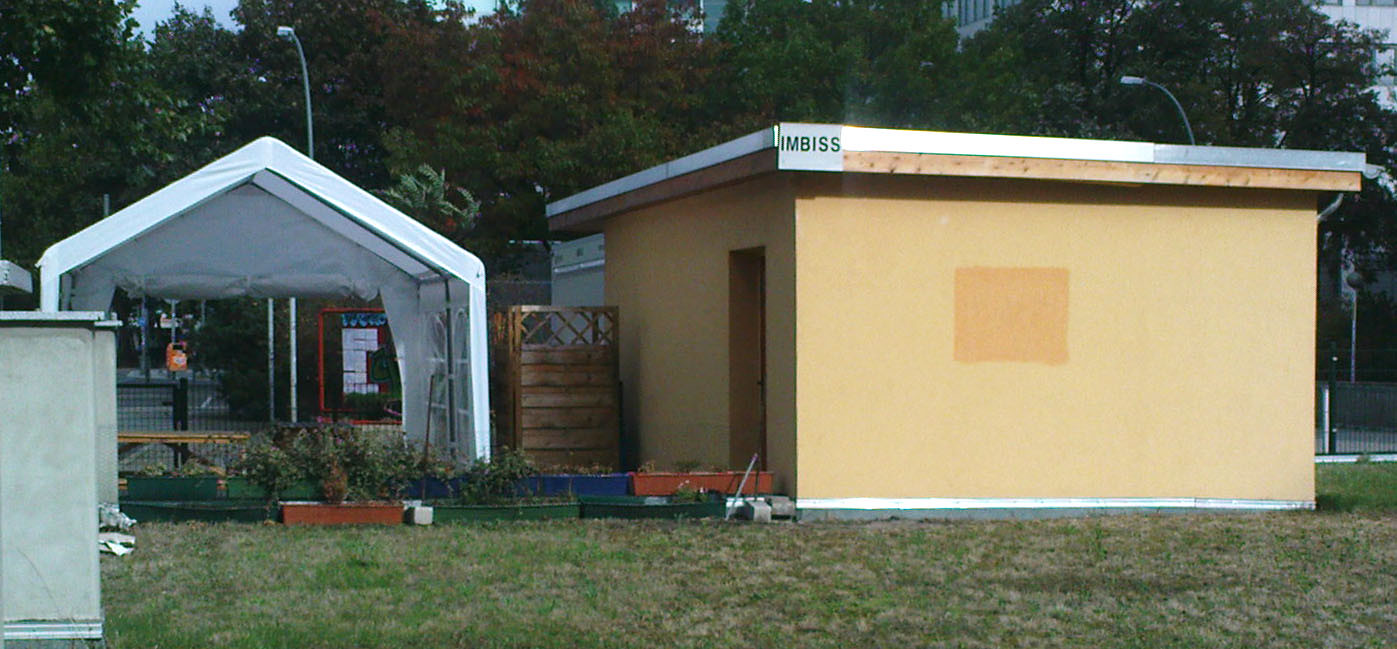This image depicts a square, yellowish-tan concrete or brick building with a flat, tin-covered wooden roof, positioned on a patchy grassy lawn area that appears to be the front yard of the structure. The upper corner of the building features a white sign with the text "I.M.B.I.S.S.," indicating it might serve as a place where people can get a meal or snack. To the left of the building stands a large wooden lattice and an open tent area, reminiscent of a reception tent used at outdoor weddings, with benches likely placed underneath for seating. 

Numerous potted plants arranged in green and tan (or orange-ish) planter boxes line the grassy area in front of the building. The planters are neatly organized, with several green planters and a single tan one interrupting the sequence. 

In the background, the scene extends to show a collection of trees, behind which taller urban buildings and street lights can be seen, hinting at a city setting. Additionally, there is a black metal gate enclosing this entire grassy area, suggesting it is an official or semi-private space, possibly with restricted access. Finally, elements such as gardening tools scattered around imply an active gardening effort near the building.